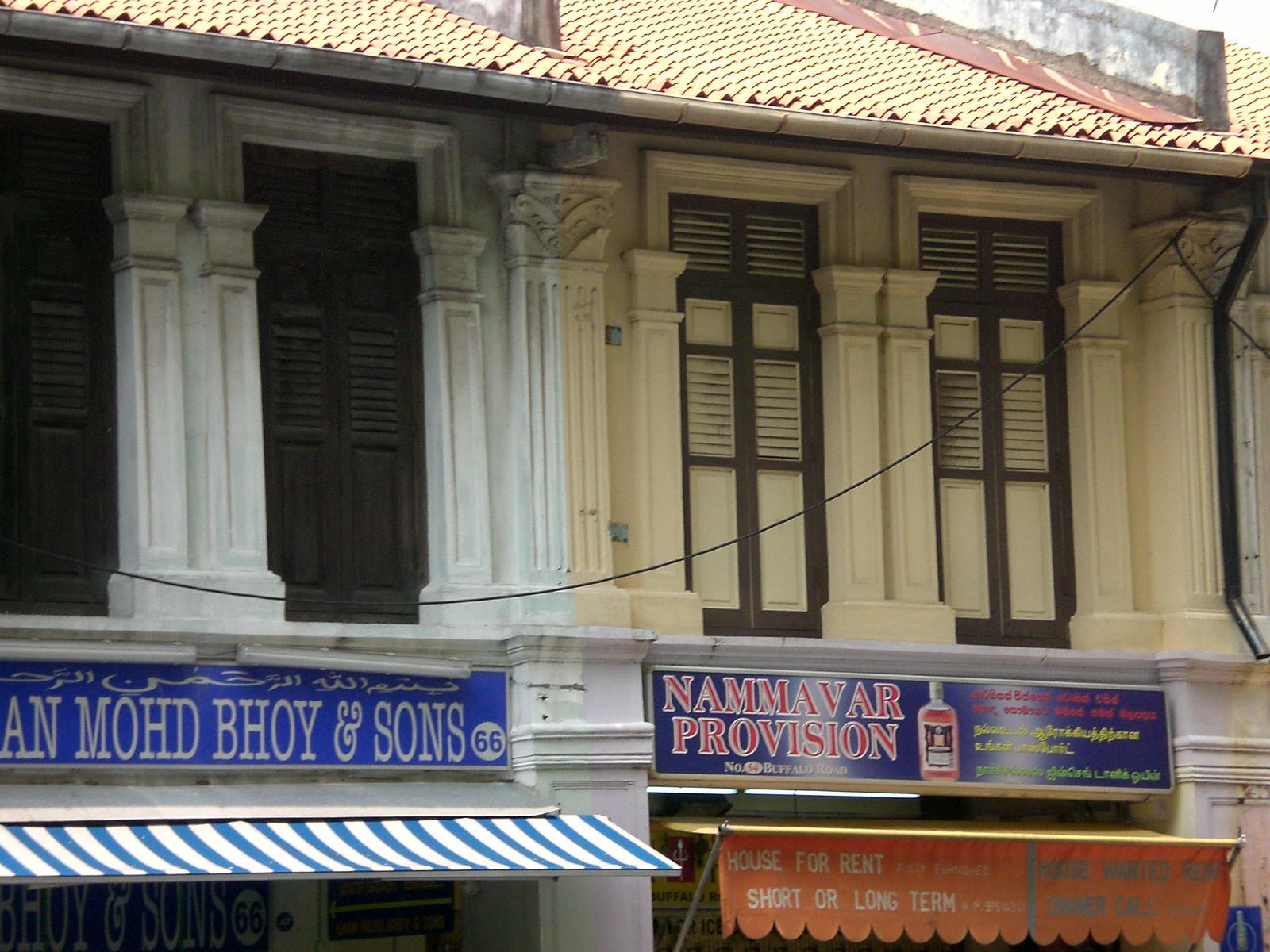The image showcases an outdoor daytime view of two adjacent commercial buildings. The building on the right is predominantly light yellow with door-shaped windows featuring blinds, and is topped with a yellow roof. An orange awning on this building displays signage in a foreign language, likely reading "Mode, Boy & Sons." Beneath this, there's additional red signage that includes a bottle graphic and the phrase "Namavar Provision," indicating a store beneath.

On the left, the other building is white and brown, with distinctive white pillars that have black shutters. It also features a blue and white striped awning with signage for "House for Rent short or long term" in an orange, shell-like banner. At the lower part of the image, the storefront signage is further detailed with various colors including red, blue, green, and gray. The buildings dominate the photograph, leaving only a sliver of sky visible at the top, suggesting the image was taken mid-day. The overall scene appears to be set in a commercial district, with the buildings occupying most of the frame and indicating a bustling area for local businesses.